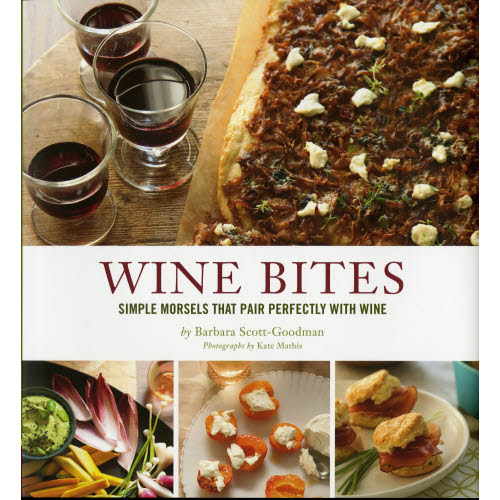The cover of the book titled "Wine Bites," features a clean white background with red text prominently displaying the title. Below the title, in black text, it reads: "Simple morsels that pair perfectly with wine," authored by Barbara Scott Goodman with photography by Kate Mathis. The upper portion of the cover, spanning about the top third, showcases a row of three clear glasses filled with red wine placed on a brown table. Beside these glasses, there is a piece of toasted bread, possibly focaccia, adorned with what looks like cream cheese, brown meat, white chunks of mozzarella, and green garnishes such as basil. Lower on the cover, there are three square photographs: one featuring a dish with raw vegetables and a green dip, another with strawberries and cream cheese, and the last image displaying pastries with ham and eggs. This well-curated cover image clearly suggests that the book presents an array of small dishes or "wine bites" that pair exquisitely with wine.